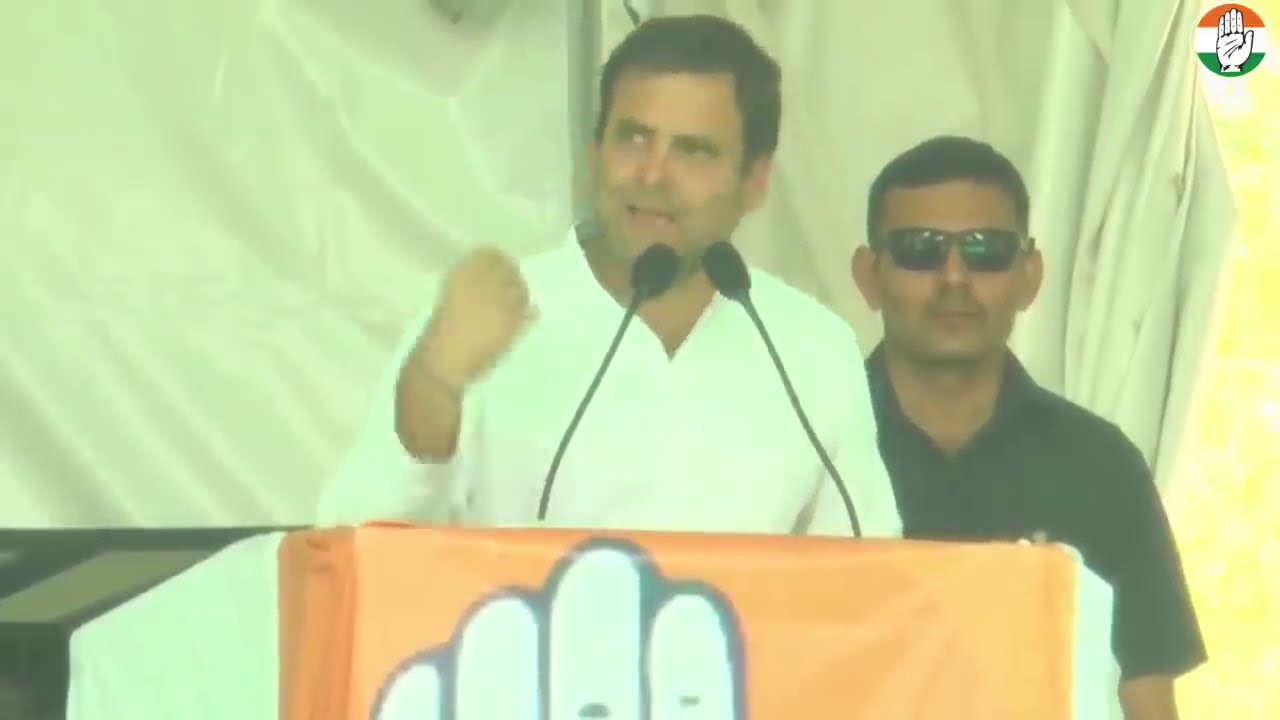In this slightly fuzzy and hazy image, two men are captured standing at a white and orange podium with two black microphones positioned around the mouth of the man speaking. The man at the podium, centered in the image, is wearing a white long-sleeved v-neck shirt. He has slicked-over brown hair, a fair skin complexion, and a non-smiling, somewhat grim expression as he looks to his right. His right hand is raised toward his shoulder in a closed fist. To his left, over his shoulder, stands a man who appears to be a bodyguard, with short black hair, a fair skin complexion, black sunglasses, and a black short-sleeved polo shirt. In the top right corner of the image is a notable icon of a hand with five fingers, palm facing forward, set against the colors of the Indian flag – orange, white, and green. The backdrop behind them is a light sea green curtain, adding a soft, neutral tone to the setting, which captures a moment of the man giving a speech.